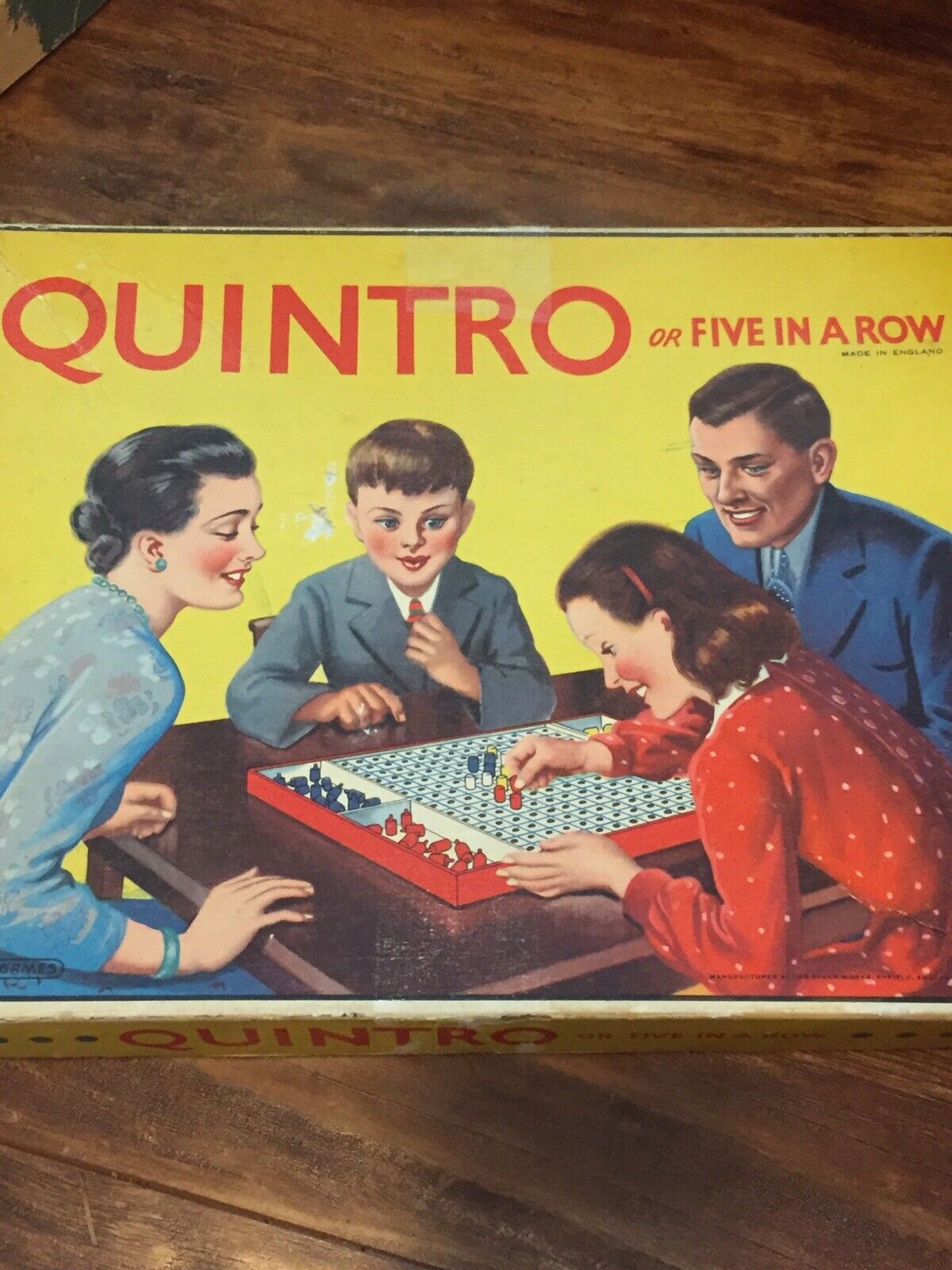This is a detailed photograph of a classic board game box for "Quintro," prominently set against a yellow background. The box displays "QUINTRO" in bold, capital red letters at the top left, followed by "Or, five in a row" in smaller text, with "Made in England" subtly printed in black underneath. The box art depicts an illustrated 1950s-style family of four engrossed in the game: the mother in a light blue dress with a blue bracelet, the father in a blue suit, the daughter in a red dress with brown hair, and the young son in a gray suit. The daughter is shown inserting a red piece into the game board while the rest of the family watches. This actual game box rests on a brown wooden table, mirroring the table depicted in the illustration where the family is seated, enhancing the nostalgic and authentic feel of the scene.